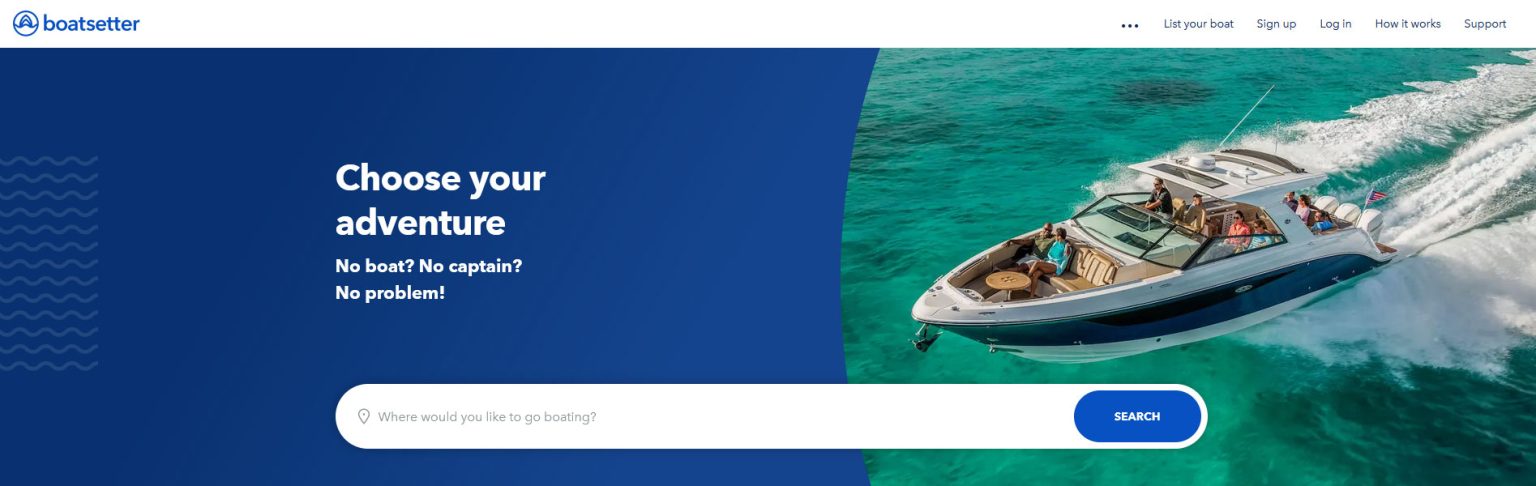This image is a screenshot of a simplistic web page design. The page is segmented into a few distinct sections: 

At the very top, there's a white navigation bar spanning the width of the page. In the upper right corner of this bar, several clickable options are listed sequentially: "Use Your Boat," "Sign Up," "Log In," "How It Works," and "Support." Adjacent to these options, three horizontal black dots are aligned vertically, possibly indicating a dropdown menu or additional options.

In the upper left corner of the navigation bar, there is a recognizable website icon. Next to the icon, the text "Boat Setter" is displayed in a blue font. To the left of this text, there is a small circular icon containing an upside-down 'D', which appears to be blue as well.

Below the navigation bar, the main content is divided into two sections within a rectangular frame. On the left side, the background is purple and features white text that reads: "Choose Your Adventure. No boat. No captain. No problem."

On the right side of this rectangular frame, there is an image depicting a small white boat with a blue stripe navigating through a body of water, either an ocean or a lake. The boat is moving to the left. On the deck, two people are romantically interacting, while a man is seen steering the vessel.

The blog page combines practical navigation options with an inviting visual and textual call to action, effectively encouraging users to explore boating adventures even if they lack personal boating resources.